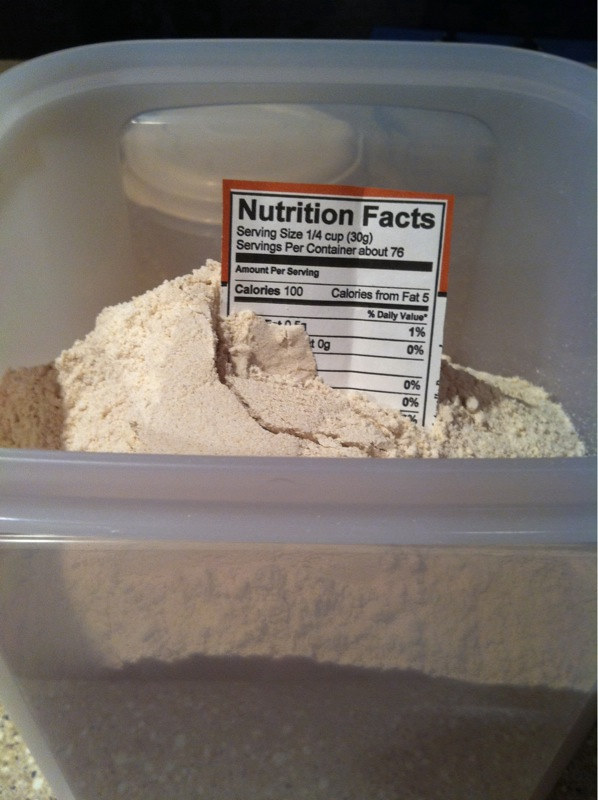The image features a close-up view of a Tupperware container filled with a powdered substance. Innocently peeking out from the middle of the powder is a cut-out segment of nutritional information, presumably sliced from the side of the original packaging box. The powder, once contained within the box, has clearly been transferred to the Tupperware for storage. The photograph is taken from a top-down perspective, providing a clear and detailed look at both the powder and the protruding nutritional facts cut-out.